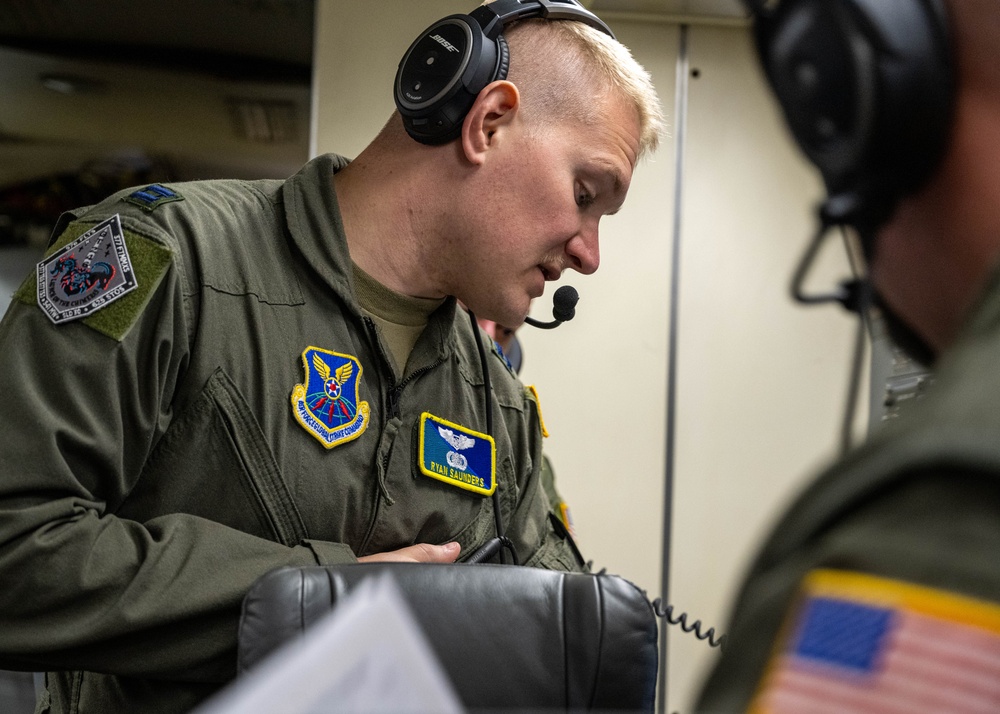In this detailed indoor photograph, two men in military uniforms are captured, with the primary focus on the man in the background, Ryan Sanders. Both men are outfitted in khaki-green jumpsuits adorned with multiple patches, including a recognizable American flag on the man in the foreground's shoulder, partially visible as he stands slightly out of focus to the right. The primary subject, Ryan Sanders, is clearly visible and in sharp focus. He has blonde hair and wears over-the-ear Bose headsets with a boom mic positioned near his mouth. For a better auditory awareness, he has pulled the headphone back slightly to free one ear. His jumpsuit features a blue badge on his chest with his name, "Ryan Sanders," embroidered in yellow letters, and another patch with wings. In his hand, partially obscured by a chair, he holds an object connected by a coiled wire, likely a microphone. The scene captures a moment of attentive communication, emphasizing the detailed and disciplined appearance of the military personnel.